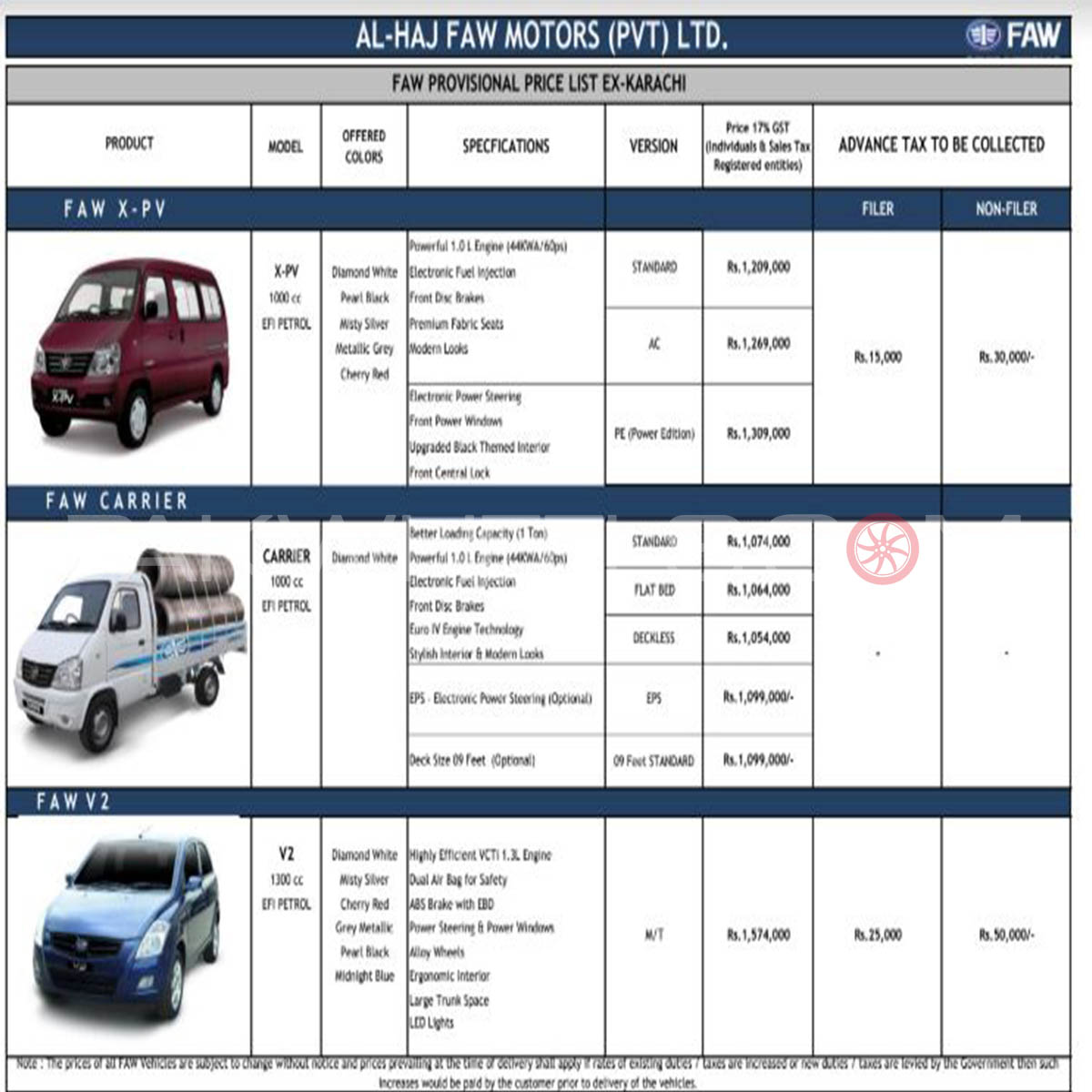This image displays a detailed section of the Al-Haj Faw Motors PVT Limited website. The top header features a blue background with white text, prominently showing the company's name. Situated in the upper right corner is a logo in white and blue, accompanied by the text "Fah."

Beneath the header, the site lists the "Provisional Price List X Karachi." This section organizes information into columns with the following headings from left to right: Product, Model, Offered Colors, Specifications, Version, Price, 17% GST, and Advanced Tax to be Collected. Although some text is blurry, the general structure is discernible.

The first product listed is the XP4 or XPV, available in Diamond White, Pearl Black, Misty Silver, Metallic Gray, and Cherry Red. This model’s version is specified as Standard with AC and PE.

Below that, the Fah Carrier is mentioned, offered solely in Diamond White.

Lastly, the Fah V2 is showcased with color options including Diamond White, Misty Silver, Cherry Red, Gray Metallic, Pearl Black, and Midnight Blue.